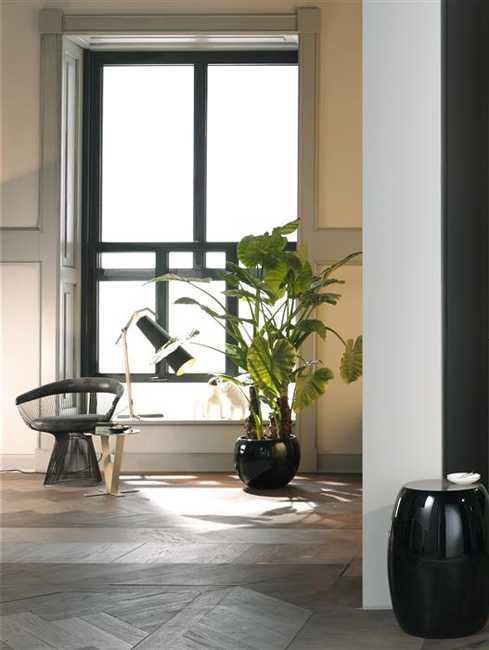This color photograph, taken indoors during the daytime, likely depicts a minimalist living or sitting room with a modern aesthetic. The room features light wooden floors, white walls, and gray molding. A large window with black frames is partially open, allowing ample daylight to illuminate the space. On the left side, a short black wire chair sits next to a sleek black lamp. Adjacent to the chair is a substantial black pot holding a tall, lush green plant with large leaves, approximately three feet tall. To the right, there's a small round black table, on which rests a white object that could be an ashtray. Additionally, a light brown table or stand is visible at the bottom right of the image. The room's décor is both functional and stylish, characterized by its clean lines and contemporary furnishings.